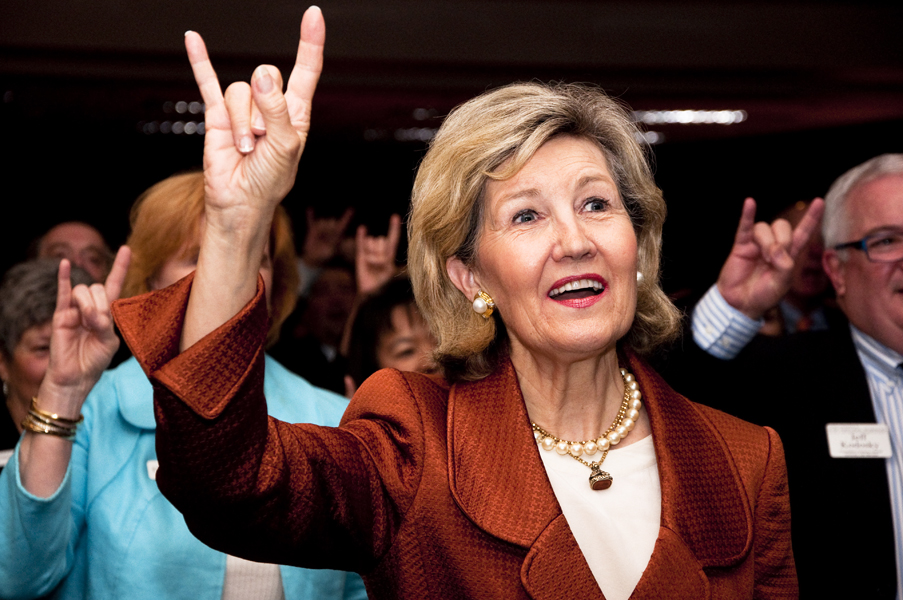The photo depicts a group of older adults, likely aged 60 and above, all raising their right hands with their pinky and index fingers extended, middle fingers folded down and held in place by the thumb, forming a distinctive hand sign. At the forefront is a woman dressed in a rust-colored business jacket, a white shirt, and adorned with a pearl necklace as well as some gold jewelry. Her light brown hair features highlights, and she is smiling with a slightly open mouth. To her right, a man in a suit and glasses mirrors the same hand gesture. In the background, both men and women, including a woman in an aqua blazer, also participate in this synchronized sign, which might be the Texas Longhorns "hook 'em" signal or potentially a different symbol. The setting feels reminiscent of a political convention, possibly Republican, although the exact context and identity of the individuals remain uncertain.